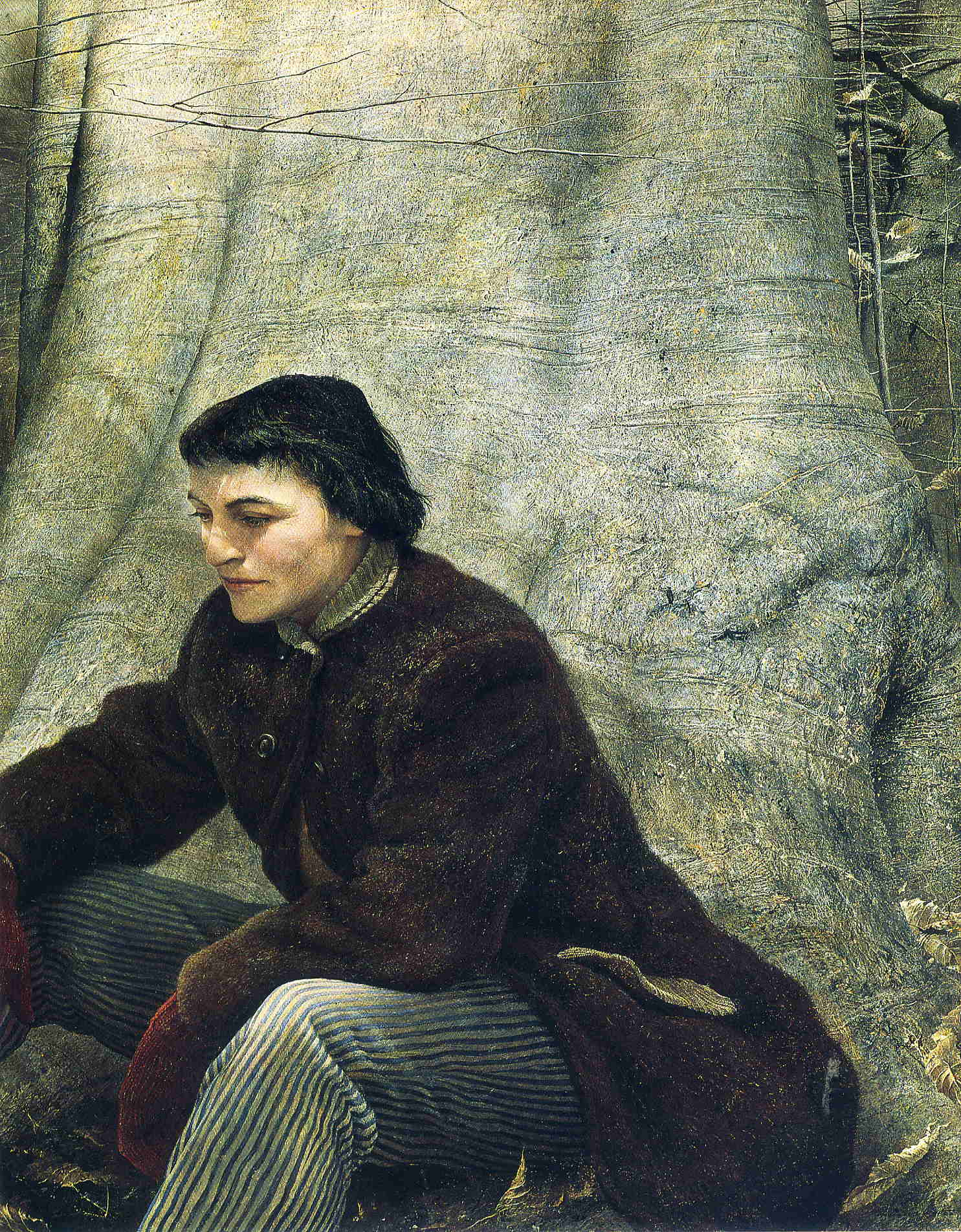The painting depicts a somber-looking person, likely a woman in her twenties to mid-thirties, sitting near the base of a large tree. The individual is dressed in a combination of rough, layered clothing, including a thick, ragged brown coat and visible underneath a jacket. They have on red mittens and long blue and white striped pants. The person's short black hair is slightly curled at the top and down the sides, with crow's feet hinting at a somber, pensive expression. Their body language, with legs extending off the image and facing to the left, together with the broad, plain facial features distinguish neither strongly feminine nor masculine characteristics. The backdrop features the expansive trunk of a smooth-barked oak tree, which dominates the upper portion of the vertical canvas and showcases bark of a light color. The absence of an artist’s signature or accompanying text in muted grayscale tones, possibly interspersed with beige and olive green hues, gives the piece its stark and contemplative atmosphere.